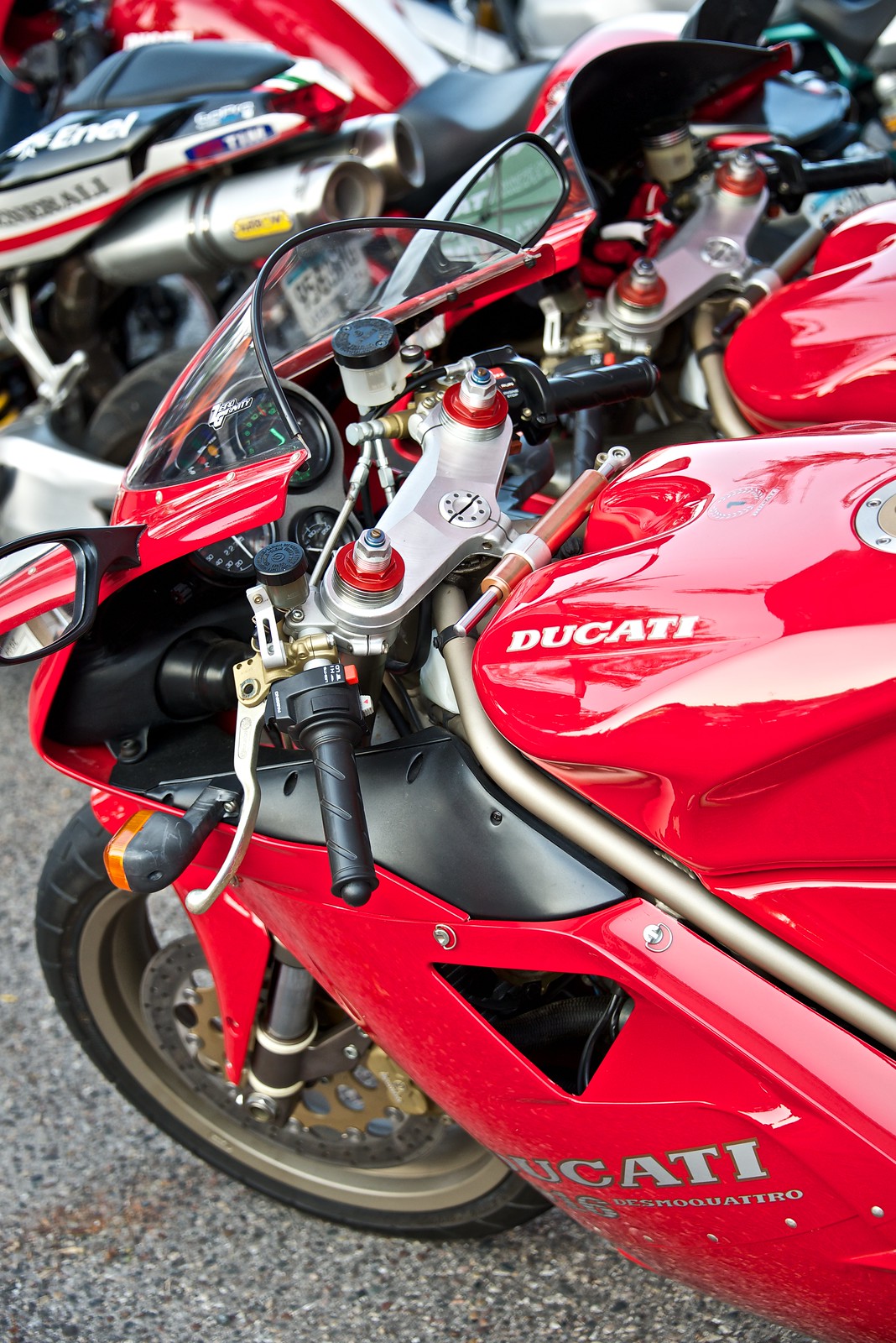The image features a close-up of a lineup of red Ducati sports bikes parked on a tar or gravel surface. The foremost bike, prominently positioned at the center and slightly angled to the left, showcases intricate details such as the Ducati logo in white on the body, the fuel tank, the handlebars, the instrumentation console, and the windscreen. Despite the partial view that cuts off part of the motorcycle, elements like the gears, clutch handles, speed, and fuel meters are clearly visible. In the background, more Ducati bikes can be seen, also pointed to the left but slightly blurred with a bokeh effect, giving a sense of depth. Visible parts such as tires, silencers, black seats, mirrors, and headlights contribute to the composition. The image is predominantly colored in shades of red, black, gray, and white, with minor accents of orange and yellow.